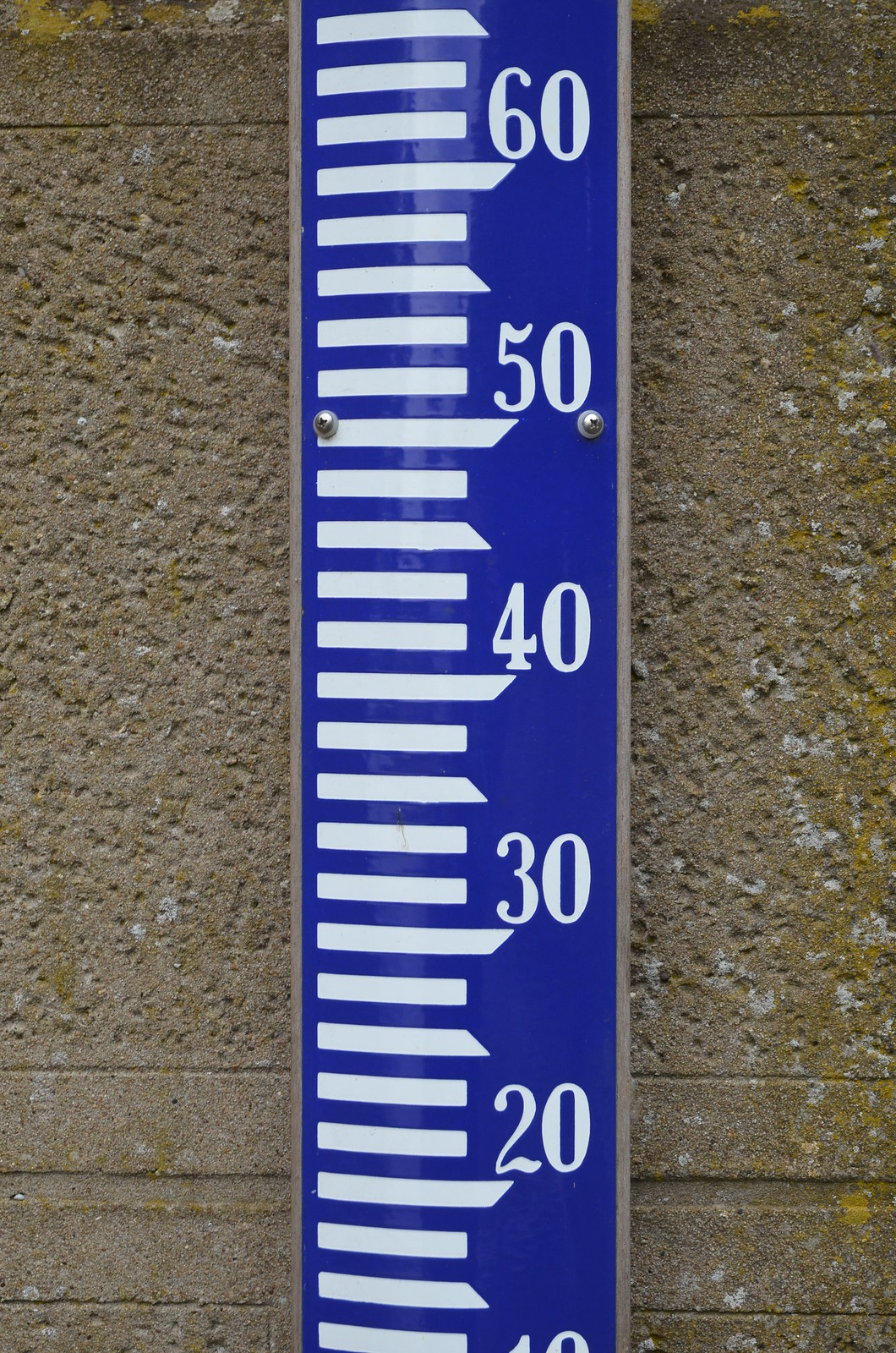The image showcases an exterior concrete wall characterized by its textured surface, accentuated with natural growth resembling moss. The concrete is marked with various divots and depressions, lending it an aged appearance. A distinctive blue measuring stick, likely intended for gauging height in inches or similar units, is the central focus. The ruler-like device is securely fastened to the wall with two screws, positioned just below the 50-inch mark. The visible segments of the measuring stick bear clearly printed numbers starting from 20 at the bottom and continuing through 30, 40, 50, and ending slightly above 60. The number 10 is partially obscured, suggesting the measuring stick starts slightly below the frame of the image. There is a faint horizontal line near the base of the wall. This entire setup suggests a practical, outdoor utility for precise measurements.